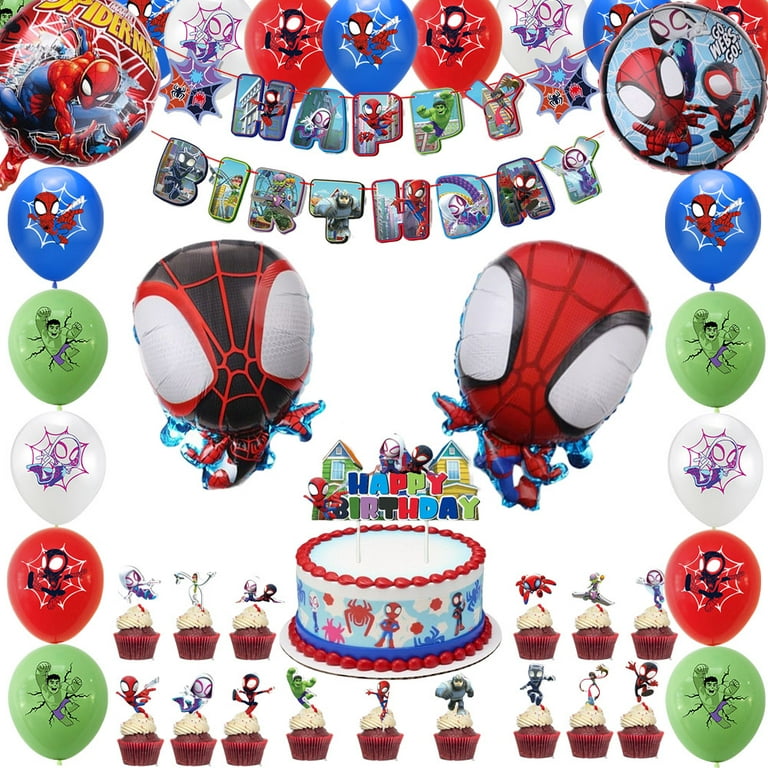The image depicts a vibrant and busy birthday-themed scene centered around Spider-Man and other comic book characters. At the top, there is a series of Mylar balloons featuring different versions of Spider-Man in red, white, and blue colors, some with Spider-Man in action poses and others showcasing his iconic web patterns. Just below this row, there are two banners made up of balloon letters spelling out "Happy Birthday," with each letter adorned by youthful versions of superheroes like Spider-Man and the Hulk.

In the middle section, two large Mylar balloons also showcase Spider-Man in different costumes, one red and one blue, adding to the celebratory atmosphere. Below the banners, there's an eye-catching red, white, and blue Spider-Man-themed birthday cake, decorated with spider decals and an inserted "Happy Birthday" graphic. Flanking the cake are rows of cupcakes in red wrappers, topped with Spider-Man and Hulk-themed decorations.

The sides of the image are bordered with a mix of colorful balloons—blue, green, white, and red—each featuring decals of Spider-Man and other superheroes. Additional circular Mylar balloons featuring Spider-Man are located in the top left and top right corners, completing the festive and superhero-packed imagery.